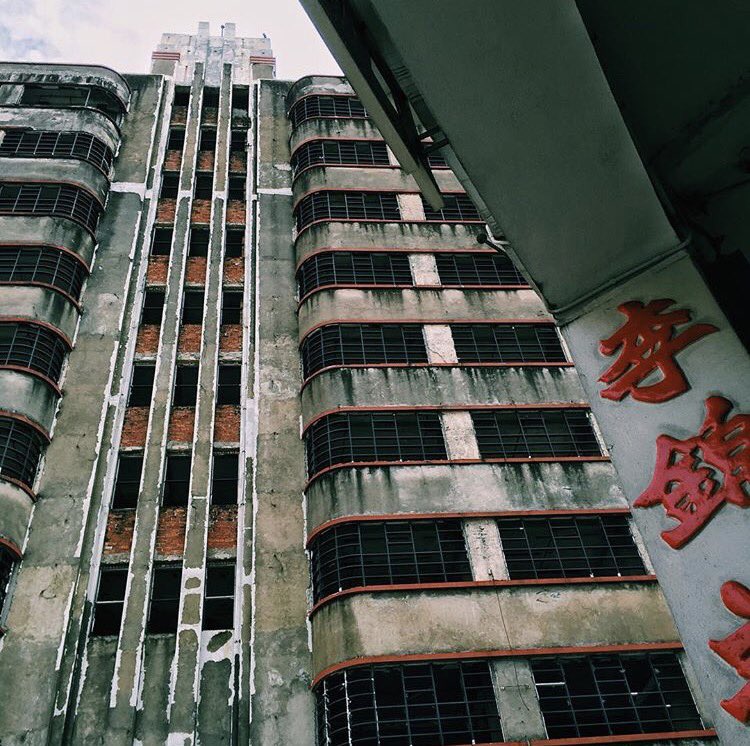This photograph captures a striking, upward view of an abandoned skyscraper, possibly located in China, that exudes an eerie, post-apocalyptic atmosphere. The building's façade, once green, is now largely stripped to bare stone, giving it a gritty grayish-green appearance with dark streaks from recent rain. The eight-story structure features two columns of bay lobby windows flanking a central column adorned with three smaller windows running vertically.

Flanking either side of the building are almost cage-like structures, adding to its dilapidated feel. In the foreground, a doorway or wall of a nearby building is partially visible, adorned with red kanji characters that are intricately carved into the stone and remain perfectly intact, juxtaposing the decay of the main building. Most of the kanji characters are cropped out of the frame, but the first character is visible along the very edge of the photograph.